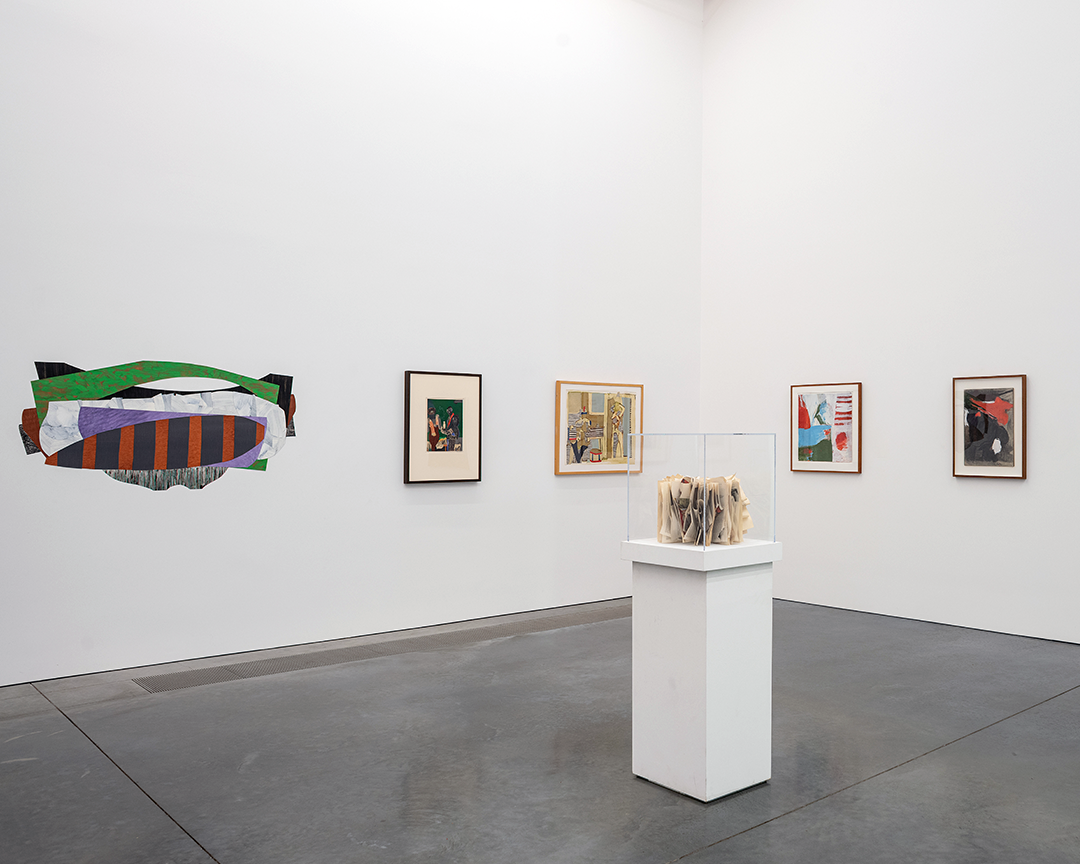The image depicts a museum art exhibit with a large, empty space characterized by plain gray floors and very high, stark white walls. The walls extend out of frame, leaving the ceiling unseen. Central in the room is a white pedestal capped with a clear glass box containing what appears to be an art piece composed of layered or possibly crumpled papers standing upright, suggesting significance. On the walls are four framed artworks—two on the right wall and two on the left—each showcasing pictures or illustrations. Additionally, on the leftmost side of the left wall, there is a vibrant, multi-colored, striped painting featuring a combination of orange, blue, green, white, and purple stripes.